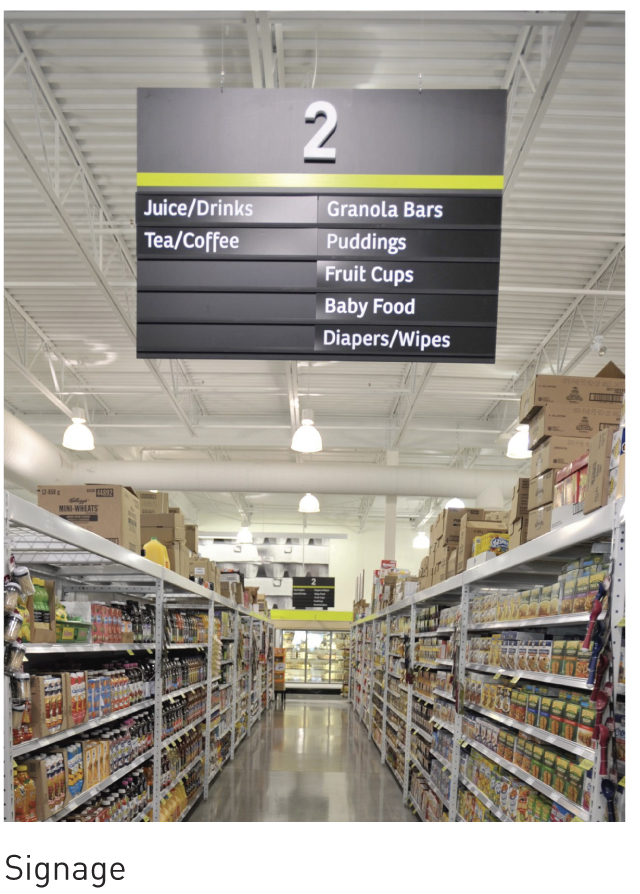The image is a color photograph in portrait orientation, capturing a meticulously clean and polished aisle in a grocery store. The photograph's perspective leads the eye down the aisle, which ultimately vanishes into what appears to be a refrigerated or freezer section at the back of the store. The highly reflective concrete floor is both spotless and gleaming.

On either side of the aisle, shelves are neatly stocked with products, stretching out and converging toward the center of the image, enhancing the sense of depth. The ceiling, which is visible above, is constructed of corrugated metal painted white, giving the interior a modern industrial look. Illumination is provided by lights hanging from the ceiling. These lights are uniquely shaped, resembling street lights but equipped with fluorescent bulbs, contributing to the well-lit environment.

Prominently hanging from the ceiling is a brown or black signage indicating this is aisle number 2. The sign features a large white numeral "2" at the top, followed by a yellow stripe. Beneath this stripe, the sign is divided into five slots or sections designed to hold interchangeable labels. The current labels on the sign include (in order from left to right): "juice/drinks," "granola bars," "tea/coffee," "puddings," "fruit cups," "baby food," and "diapers/wipes." Interesting to note, the labels are configured such that "juice/drinks" and "tea/coffee" occupy the left side with three slots still available below them, while the remainder of the labels fill up the right side entirely.

This well-organized and vibrant image captures the essence of a clean and modern grocery store aisle, with clearly marked signage aiding shoppers in finding their desired products.